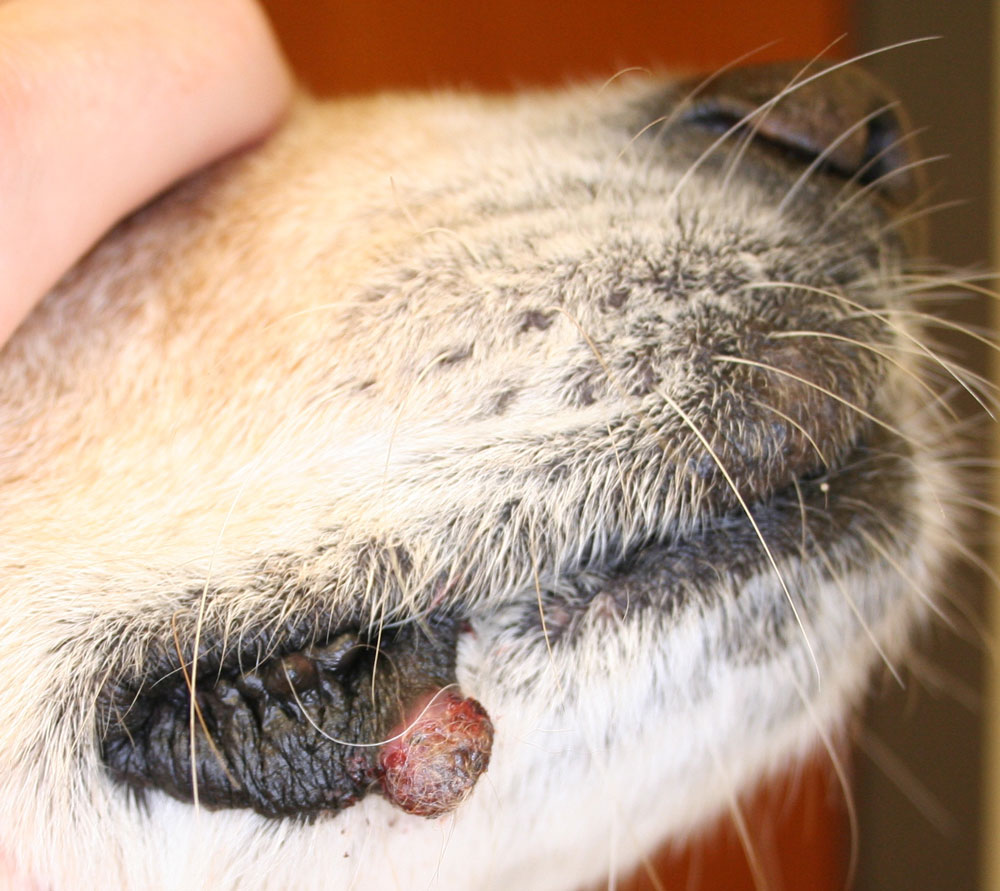This color image is a highly detailed close-up shot of a dog's mouth, focusing on a distinct growth. The dog's muzzle features a palette of white, gray, and light blonde fur, with very small whiskers jutting in various directions. Its black nose is prominently visible, alongside black lips adorned with an unsettling reddish growth that spans from pink to darker reds and blacks, with some sections appearing to have fur. The image also includes part of a human hand in the upper left corner, suggesting someone is holding the dog’s muzzle to better capture the shot. The background is blurry with warm wooden and gray tones, emphasizing the prominence of the dog's muzzle and the concerning growth.